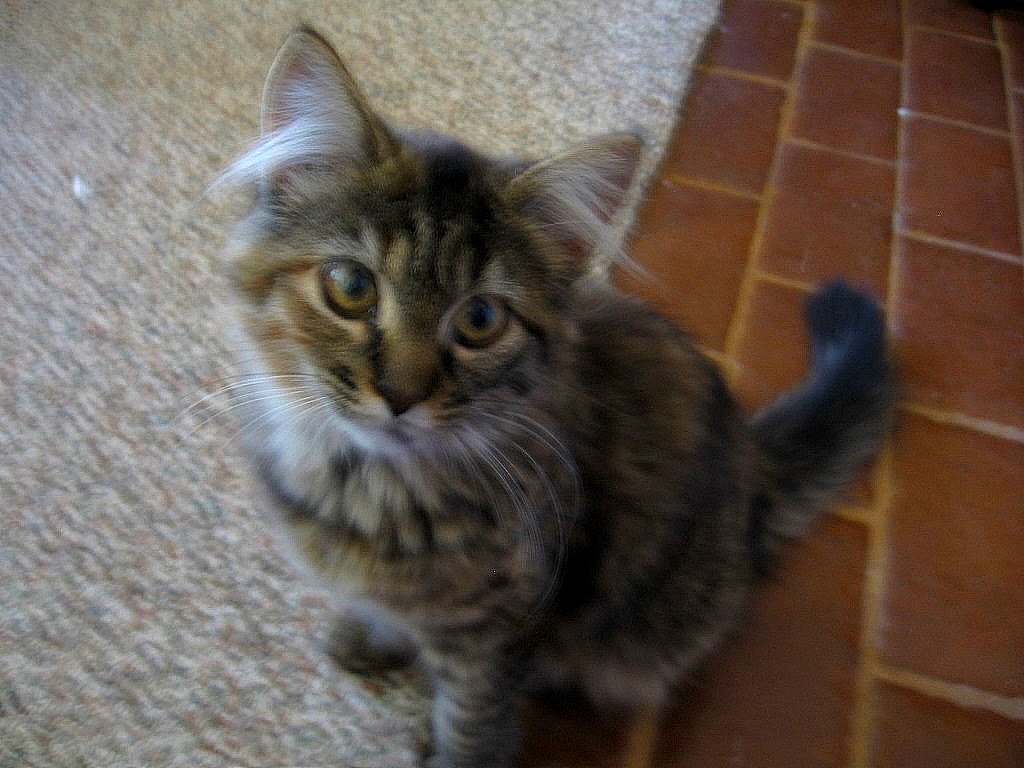The image depicts a tabby cat with predominantly brown and gray fur, interspersed with black stripes, and a slight thick hair texture. This cat has distinctive white fur tufts protruding from its ears, a brown nose, and a touch of white around its mouth. Its captivating golden eyes are fixed directly at the camera as it sits poised in a likely indoor setting, possibly a living room. The cat is centered in the photograph, with half of its body resting on a gray Berber carpet, while its tail extends onto what appears to be red brick flooring. This juxtaposition suggests the presence of either a fireplace or an entryway nearby. The image, lacking any text and being somewhat blurry, captures the cat’s serene yet attentive demeanor.